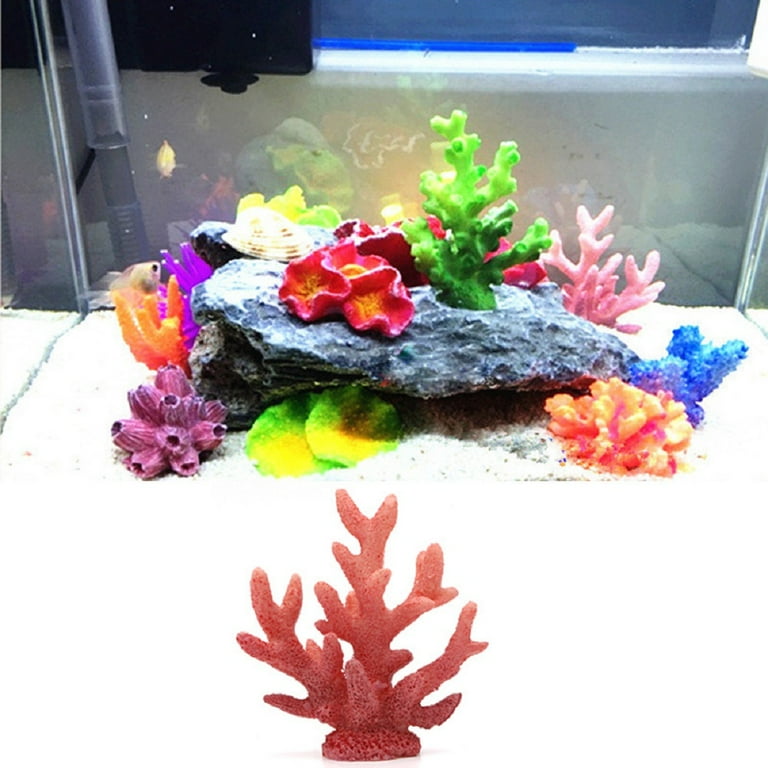The image is a detailed, vibrant snapshot of an aquarium scene, showcasing an array of brightly colored coral pieces in hues of green, pink, blue, purple, and orange. The centerpiece is a large, long, and mostly flat craggy black rock, which is surrounded by both sand and flat green objects. This rock lies on the aquarium floor and has a distinctly rugged left side. Two tiny fish can be seen peeking out from behind the coral, adding life to the underwater scene.

In the foreground, there's what appears to be a separate piece of reddish-orange, branch-like fake coral, which seems to be outside of the aquarium due to the way the photo is cropped. The dark background contrasts with the vividly lit coral and rock, likely illuminated by aquarium lighting. The glass of the aquarium reflects parts of the scene, enhancing the depth of the aquatic display. Note that the frame of the photo also includes a second image, which is a close-up of the singular reddish-orange coral piece, emphasizing its intricate, branching structure.